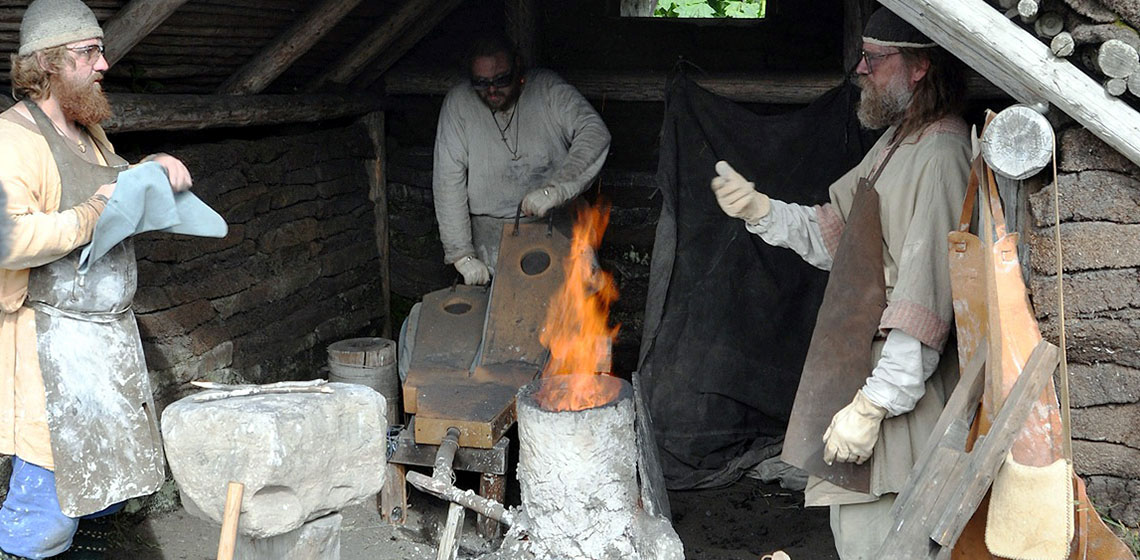In this detailed, up-close photo, three white gentlemen, who appear to be blacksmiths, are diligently working in a primitive brick and wooden forge. At the center of the image, a roaring, tall orange flame emerges from a stone fireplace, suggesting active metalworking. 

The man on the left, with brown hair, glasses, and a big beard, wears a brown apron covered in cement powder and has a yellow shirt on underneath. He also appears to be wearing blue jeans with boots and a knit cap. He is cleaning his hands with a rag.

The man in the middle, positioned slightly to the back and more shadowed due to the limited natural light filtering in, is operating a wooden bellows tool to pump air into the fire, making it roar. He is wearing a gray shirt. 

The man on the right, also bearded with some gray in his hair, wears a grayish felt covering over a white shirt, an apron, and yellow gloves. All three men's clothes are dusted with powder from their work. The interior of the hut-like forge, with its brick and wood structure, adds a rustic atmosphere to their intense, hands-on labor.